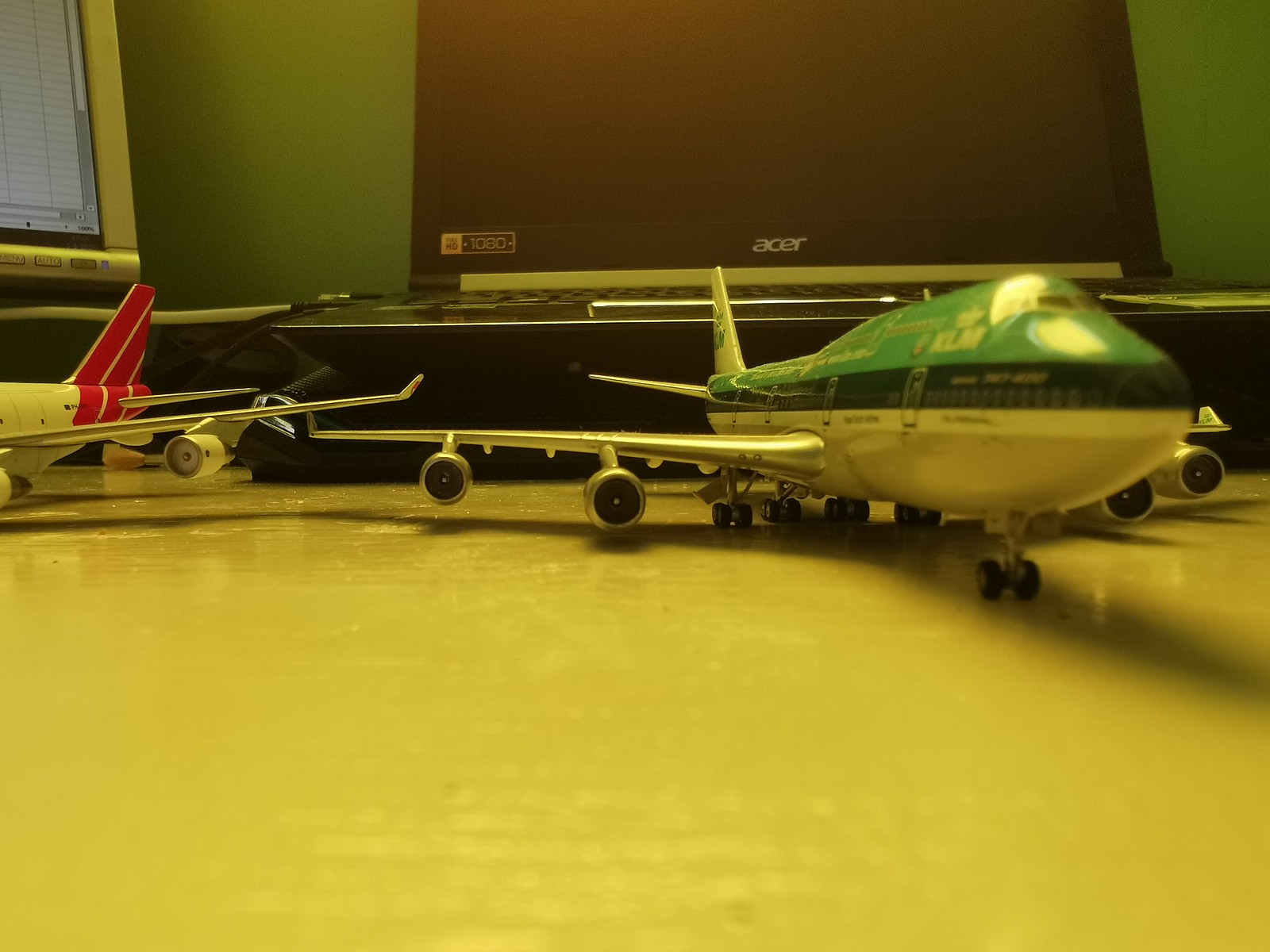This image captures a detailed close-up of a hobbyist's or boy's room, featuring a meticulously arranged scene on a shiny, gold-painted table. The table showcases two intricately designed toy model airplanes, made of metal. One airplane prominently displays a green upper body with the markings "KLM," along with a white underbelly, two sets of wings and engines, and black tires. The second airplane, slightly smaller, sports a red-striped tail and an ivory-colored body, also equipped with black tires and additional indistinguishable markings. Positioned behind these model airplanes is an open Acer laptop featuring a partially visible keyboard and a dark brown screen. The laptop is situated slightly to the right of another monitor that is also visible in the background. The overall visual creates an engaging focus on the craftsmanship of the model airplanes, set against the backdrop of modern technology.